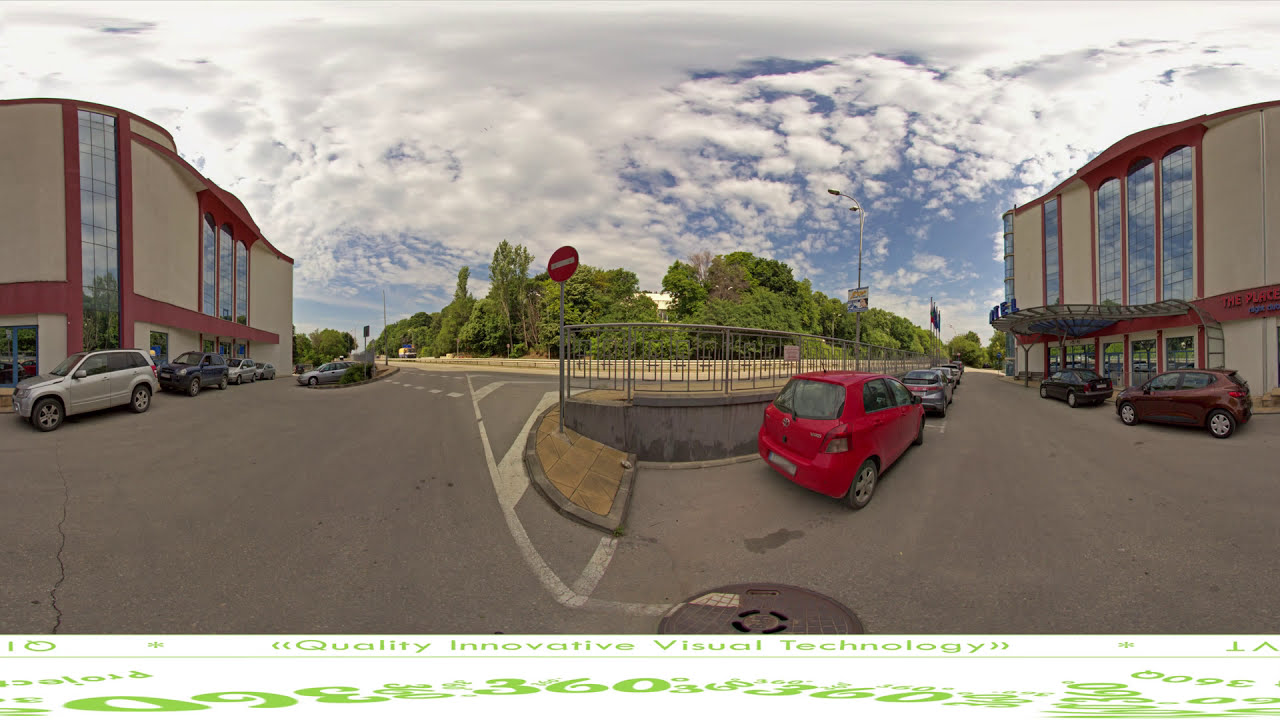The photorealistic image showcases a quiet, urban street lined with two similar two-story buildings featuring tan cement walls and rust-colored trim. These structures have tall, expansive windows stretching from the bottom to the top in various areas. The foreground reveals a gray road with white lines, and multiple cars are parked parallel to the buildings. Notably, a bright red car is parked facing three-quarters to the right near the center of the image, adjacent to a low wall that separates the buildings from the street. Behind the street, there is a lush area filled with large, dense, bright green trees. The sky is bright blue, heavily adorned with big, fluffy white clouds, suggesting an overcast yet tranquil day. Toward the right side of the image, a couple of indistinct flags can be seen in the distance, and slightly left of center is a red sign featuring a white line. The scene overall emanates calmness with no indications of any human presence or activity.